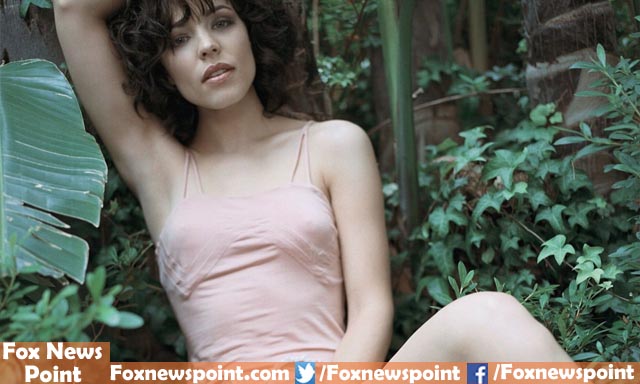In this detailed photograph, Rachel McAdams is depicted sitting outdoors in a forested area, wearing a pink camisole top and striking a relaxed yet suggestive pose. Her deep brown, curly hair falls just short of her shoulders, and she is adorned with light makeup, including lipstick, eye mascara, and painted eyebrows. She has her left arm raised above her head, revealing her underarm, while her right arm rests below her torso. Her left leg is bent, exposing her knee prominently at the right side of the image.

The background is lush with vegetation, predominantly large green leaves that resemble tropical or palm leaves, with stems and branches visible, adding to the serene and natural ambiance. The image is framed at the bottom with a transparent orange box featuring the Fox News Point banner. The banner includes text that reads "Fox News Point," "foxnewspoint.com," along with Twitter and Facebook logos followed by their respective handles. The banner is light red with white text, and it repeats the "Fox News Point" branding multiple times.

Rachel McAdams gazes directly at the viewer with a composed expression, making her the focal point amidst the earthy tones of greens, browns, and the soft hue of her pink attire.